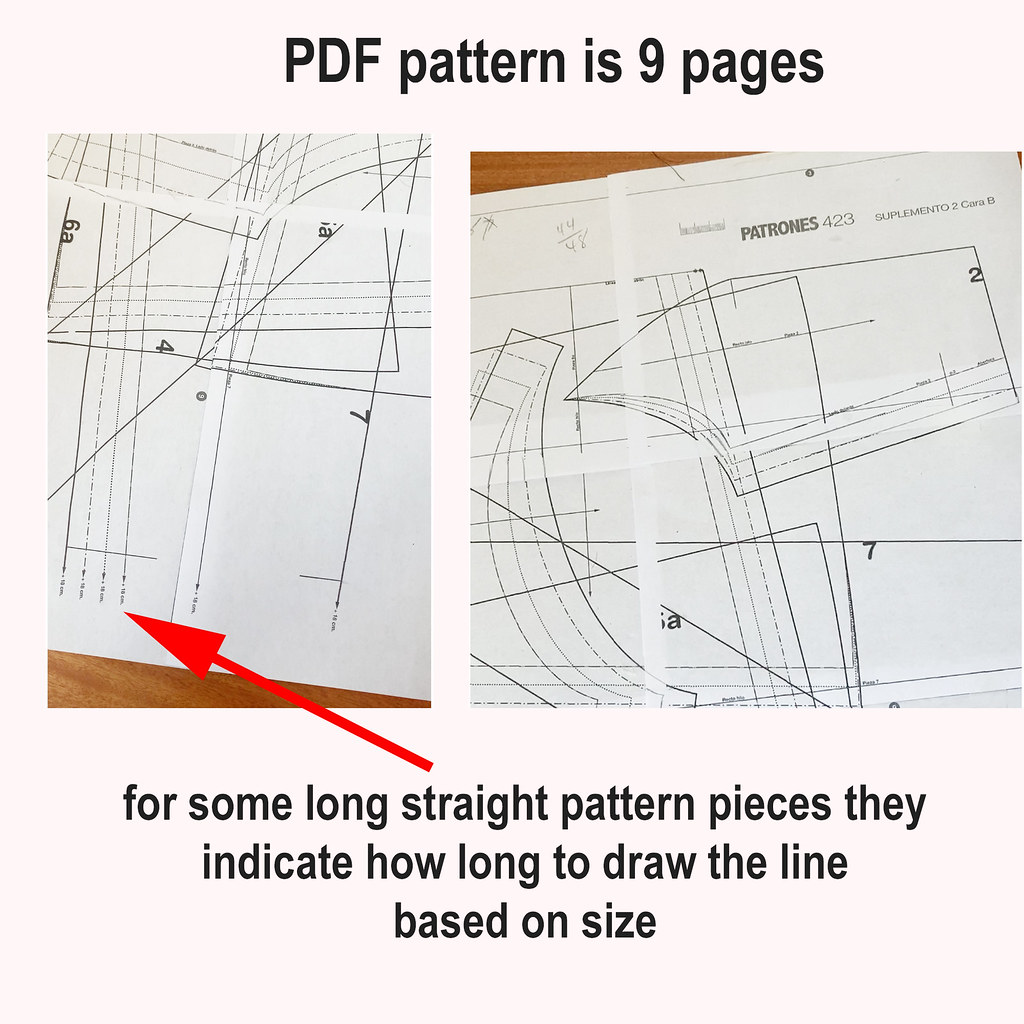The image depicts a screen grab or scan from an instructional manual with a very light pink background. At the top, clear black text reads "PDF pattern is nine pages," indicating the pattern spans nine printed pages. Below this, the center of the image features two schematic diagrams. The left diagram shows a white rectangular portrait with black lines running straight and diagonally, marked with a red arrow pointing to a particular spot. The right diagram displays a larger, enigmatic line drawing resembling a blueprint, labeled "Petronas 423" at the top. Beneath these illustrations, accompanying text reads: "For some long straight pattern pieces, they indicate how long to draw the line based on size." This page is partially placed on a wooden table, visible at the bottom of the photo. The detailed black lines and directional instructions suggest this is a detailed visual guide, possibly for assembling a pattern or design.